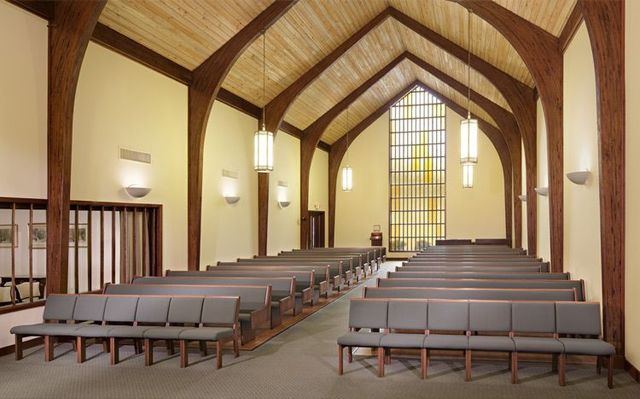This detailed photograph captures the interior of a church. The most striking feature is the A-frame ceiling made of light-colored, knotty wood, supported by five prominent black beams that arch upwards. The ceiling also hosts several long, white lights hanging down, adding to the brightness of the space. The walls of the church are off-white and include small lights along their length.

The seating arrangement consists of two long rows of light blue-gray padded chairs, aligned meticulously from the front to the back of the church. These chairs, featuring wooden brown legs, are either linked or placed very close together. Behind the chairs are additional wooden benches. The carpet beneath the chairs is light gray, but some sections reveal wooden flooring. Toward the back, there is a large, striking floor-to-ceiling window that resembles a screen design, allowing natural light to flood in.

Additionally, a door is visible on the left side, and a person can be seen standing at the very back of the church with their arms crossed. Overall, the photograph offers a serene and well-lit view of this thoughtfully designed church interior.